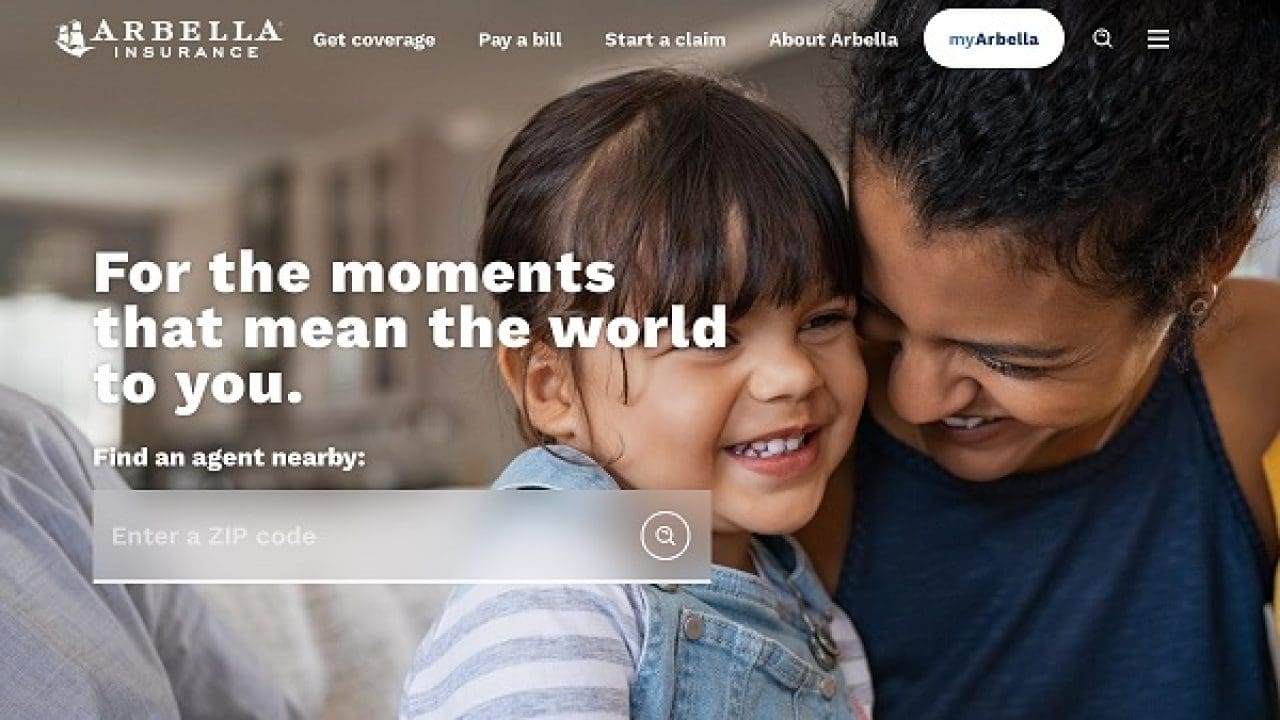The webpage features a background image of a smiling woman and her young daughter with their heads close together, creating a heartwarming visual. The woman, with dark hair, is dressed in a sleeveless blue shirt, while her daughter, also with dark hair, is wearing a gray and white striped shirt paired with light blue overalls adorned with silver buttons. 

In the upper left corner of the page, the Arbella Insurance logo, which includes a ship icon, is prominently displayed. To the right, navigation options are clearly listed: "Get Coverage," "Pay a Bill," "Start a Claim," and "About Arbella." Below these options, a white rectangular tab with curved ends is labeled "My Arbella," accompanied by a magnifying glass icon and three horizontal lines indicating the menu.

Overlaying the image in bold white text is the message: "For the moments that mean the world to you, find an agent nearby." Directly underneath, a light gray text box invites users to "Enter a zip code," accompanied by a search icon in the form of a circle with a magnifying glass inside, emphasizing the ease of finding a local insurance agent.